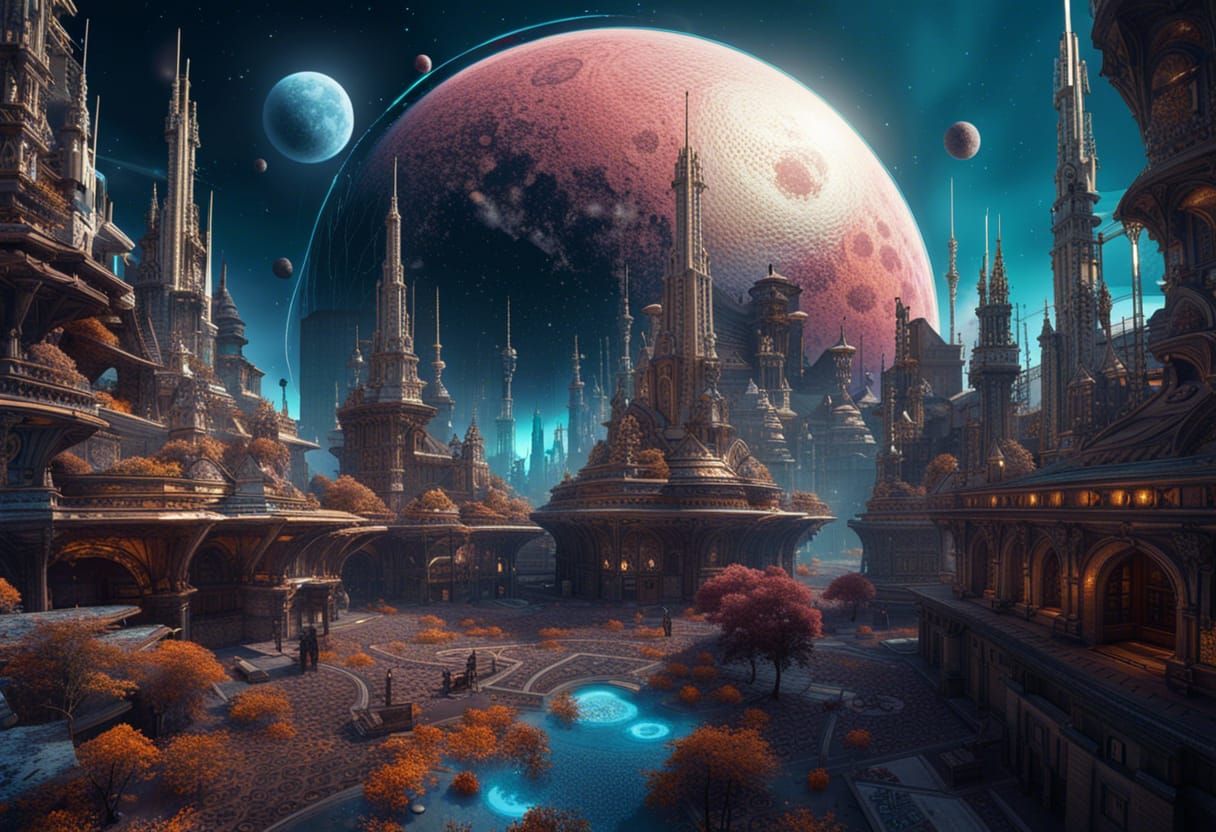The image depicts a breathtaking futuristic or fantasy cityscape on an alien planet. Dominating the sky is a massive red planet with craters, occupying nearly three-quarters of the view, accompanied by several smaller moons in shades of red and brown. To the left of this giant planet is a smaller blue moon, while a smaller brown moon can be seen on the right. The sky is densely dotted with stars and tinged with a green aurora borealis hue.

The city itself features an array of spire-like buildings with intricate engravings, their hue a blend of grayish-red and brown. These tall structures resemble the steeples of an ancient Islamic temple, exuding a majestic and otherworldly aura. Vegetation adorns the bases and decks of the edifices, adding splashes of color to the scene. Windows with lights dot the buildings, suggesting a thriving, illuminated civilization.

In the foreground, there is a serene blue pond surrounded by an orangish-red roadway or blockway, flanked by red and orange autumnal bushes and trees. The carefully arranged greenery and the small park area offer a tranquil contrast to the towering spires in the background, creating a harmonious blend of natural and architectural beauty. This striking and detailed artwork evokes a sense of wonder and grandeur, as though capturing an ancient, advanced civilization on a distant world.